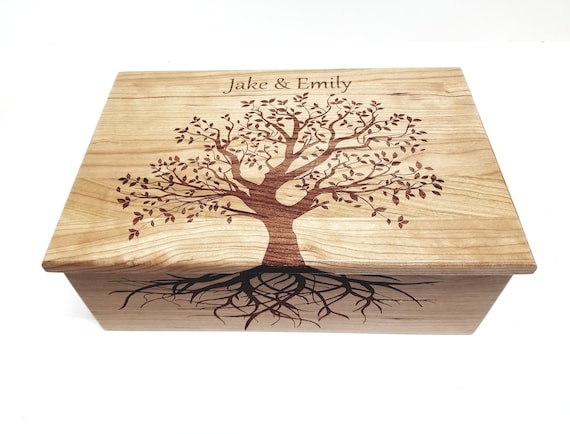This detailed image showcases a light oak, rectangular wooden memory box positioned against a white background. The box, with its visible grain details, features an intricate design of a large oak tree that appears to be burned or stained onto the wood. The tree, with a relatively short trunk, extends wide branches adorned with a mix of brown and green leaves, allowing a glimpse of the background through the sparse foliage. At the top of the box, above the tree, the names "Jake & Emily" are inscribed in script. The artistry continues as the tree's extensive, detailed roots cascade down the front side of the box, seamlessly connecting the top and front illustrations. This combination of elements suggests a deep, rooted connection, making the box an evocative keepsake piece.